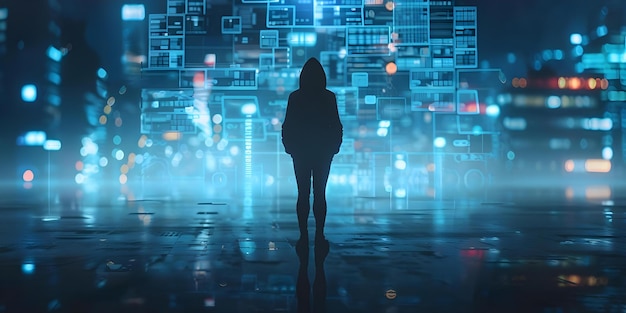In this surreal and futuristic nighttime scene, we find ourselves in an outdoor environment with a dark, uneven concrete floor scattered with puddles that reflect the surrounding lights. Central to the image is the commanding sight of stacked kitchen appliances, with washing machines occupying the bottom row and an array of miscellaneous electronics like hi-fis above them, creating an almost sculpture-like structure that dominates the background. The setting gives off an eerie blue tone, enhanced by the scattered lights of distant buildings, which add to the overall spooky atmosphere. Amidst this bizarre backdrop stands a person silhouetted against the light, draped in a black hoodie and leggings, completely shadowed and facing away from the camera. They appear to be interacting with a screen filled with boxed shapes and charts, reminiscent of data graphs, giving the scene a high-tech, hacker-room aesthetic. The blurred lights from surrounding buildings, featuring a mix of orange, white, and red hues, frame the scene with a dreamlike bokeh effect, further accentuating the mysterious and futuristic vibe.